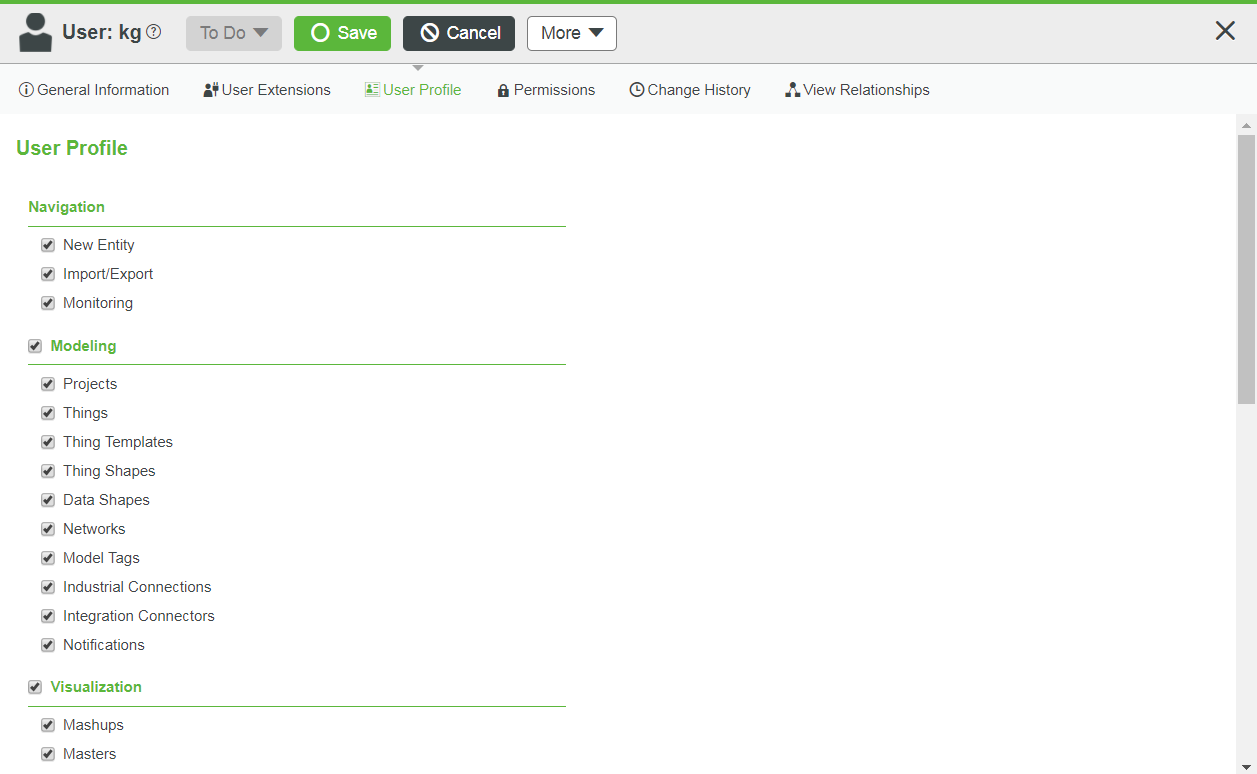The screenshot showcases an application interface, encased with a thin lime green border at the top edge. In the top left corner, there is the username "KG" displayed, signifying the current logged-in user. Adjacent to the username, four distinct buttons are placed in a row: a "To-Do Toggle" button, a "Save" button, a "Cancel" button, and a "More" button, likely providing additional options or features.

Beneath these buttons, a series of tabs are neatly arranged to offer organized navigation through various sections of the user settings. The tabs include "General Information," "User Extensions," "User Profile Permissions," "Change History," and "View Relationships."

Following this, the interface presents the user profile details for "KG" which is divided into three primary subheadings: "Navigation," "Modeling," and "Visualization." Each of these subheadings encompasses multiple configurable settings. Furthermore, every option within these categories appears enabled, indicating that all viewable options are currently activated.